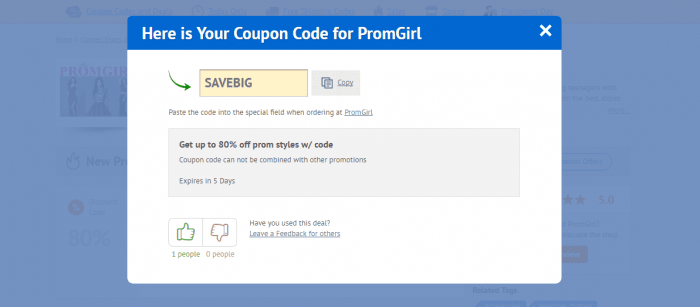The image features a prominent pop-up message displayed in front of another screen. The pop-up announces, "Here is your coupon code for PromGirl," with "PromGirl" styled as one word and the 'G' capitalized. The coupon code provided is "SaveBig," which grants users up to 80% off on prom styles. The message notes that the coupon code cannot be combined with other promotions, although parts of the text are somewhat difficult to read. Additionally, there are interactive elements within the pop-up, including a thumbs-up icon with one approval and a thumbs-down icon with zero disapprovals. In the background, there is a visible image with the PromGirl logo, indicating that the main screen belongs to a sales site. The entire setup highlights an opportunity to save money on prom-related purchases.